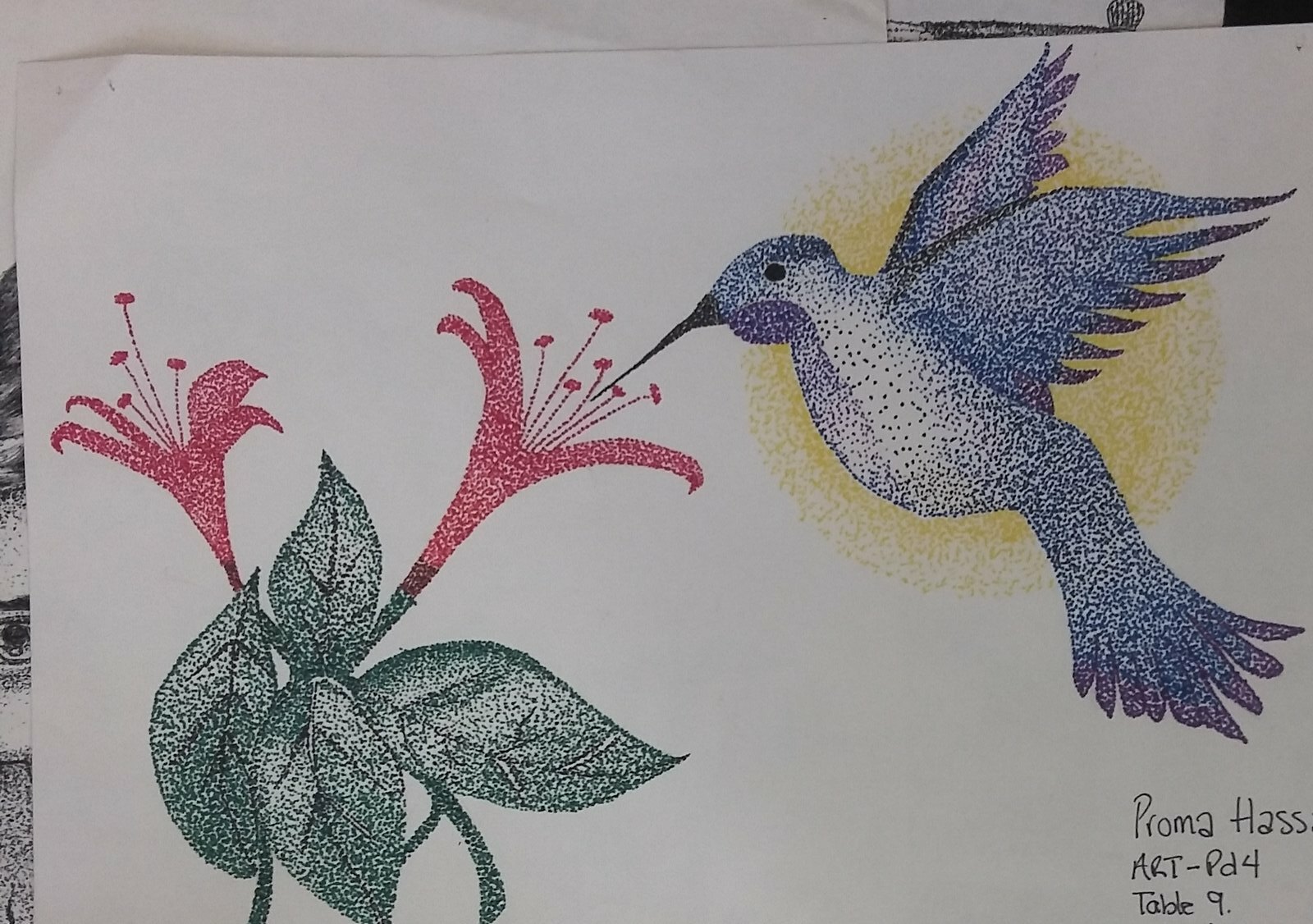In the image, the background features a muted design resembling a wife. In the bottom right corner, there is a small depiction of a house. Across the bottom, the text "art-pd4" is visible. A table with a knife placed on it occupies the lower portion, with green leaves and numerous dots scattered towards the bottom left. The top left corner showcases a flower with pink and purple-red hues. On the right side, a similar purple-red flower is present. The upper right corner is highlighted by a radiant yellow sun adorned with yellow dots. A bird is flying in front of the sun, its beak touching one of the purple-red flowers. The bird is primarily dark blue with white visible on its body and tail feathers that are dark blue tipped with white.